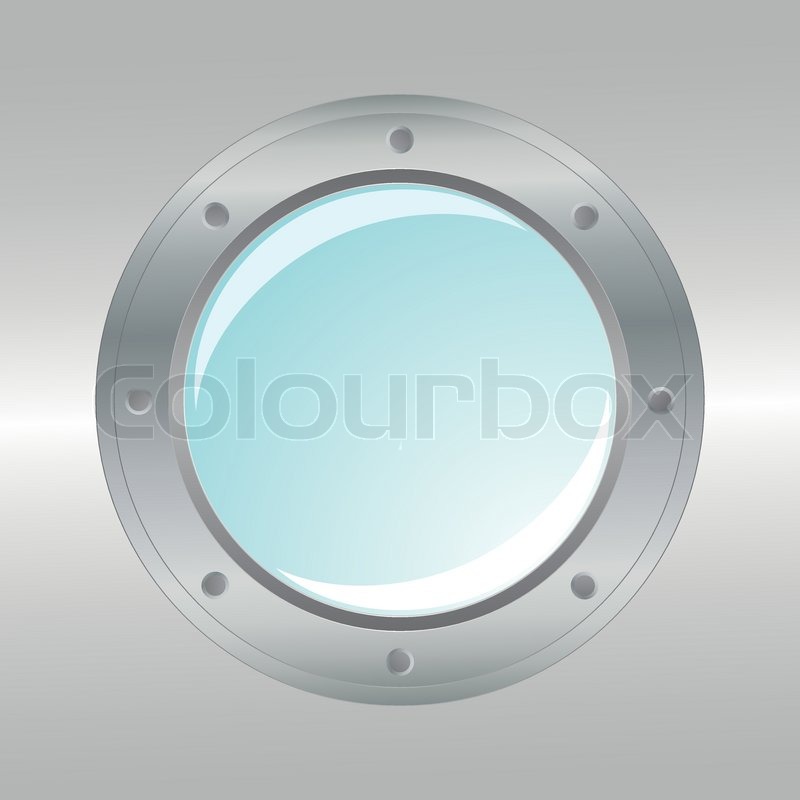The image is an animated illustration featuring a submarine's circular window. The window, framed by a grey ring with a total of 12 dark grey dots, is set against a dull silver background. The grey background appears darker at the top and bottom, with a lighter, almost white middle section that has light grey tinges. The center of the window reveals a light blue lens with swirling patterns of white. A watermark reading "COLOURBOX" overlays the window, with "colour" spelled in the UK style: C-O-L-O-U-R.